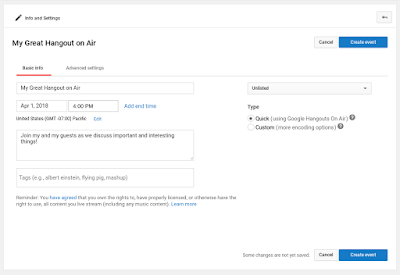Screenshot of a Device Screen Displaying an Event Creation Interface

The screenshot captures the interface of an event creation tool on a digital device. At the top of the screen, two tabs are visible: "Info" and "Settings," situated beside a black icon resembling a pen or pencil. Directly below this header, the text "My Great Hangout on Air" is prominently displayed. Underneath, navigation options reveal sections titled "Advanced Settings" and "Basic Settings," with "Basic Settings" being underlined.

The crucial event details follow. The title "My or Cat Hangout on Air" is given, alongside the date and time, "April 1st, 2018, at 4:00 PM." Below this, a blue hyperlink labeled "Add End Time" is visible, inviting further interaction.

As we move further down, two rectangular sections appear at the bottom of the screen. The first section contains the text: "Join my... Join my... Add my guest as we discuss important and interesting things." Adjacent to this is an area labeled "Tags" for tagging the event with relevant keywords.

Finally, flanking the event details are two blue buttons labeled "Create Event," located both at the bottom and the top of the screen, indicating actionable options for finalizing the event creation.